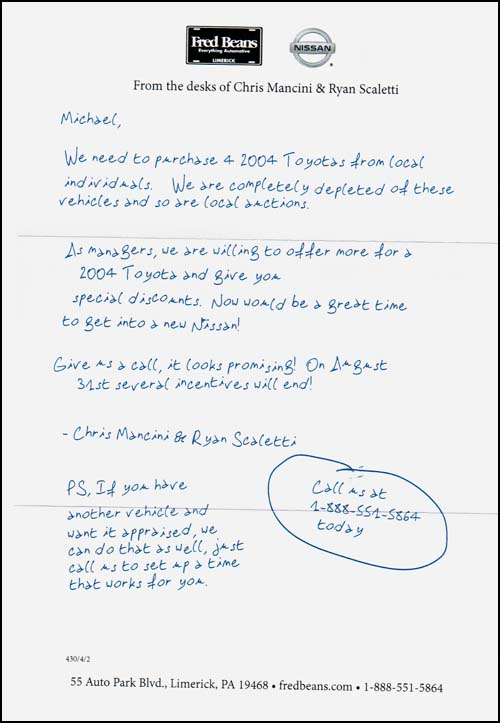This is a detailed photo of a letter on a white piece of paper with a thin black border around the edges. At the top of the letter, there are two logos: on the left, a black rectangle with "Fred Beans" in white text, and on the right, the silver circle Nissan logo with "Nissan" in the middle. Beneath these logos, the text "From the desks of Chris Mancini and Rian Scaletti" is printed in black.

Below this, the handwritten portion in blue ink begins: "Michael, we need to purchase four 2004 Toyotas from local individuals. We are completely depleted of these vehicles and so are local auctions. As managers, we are willing to offer more for a 2004 Toyota and give you special discounts. Now would be a great time to get into a new Nissan. Give me a call, it looks promising. On August 31st, several incentives will end. Chris Mancini and Rian Scaletti."

Following this, a PS note reads: “P.S. If you have another vehicle and want it appraised, we can do that as well. Just call us to set up a time that works for you.”

In the right corner of the letter, there is a circle drawn around the text "Call us at 1-888-551-5864 today."

At the bottom of the letter, the printed text reads: "55 Auto Park BLVD, Limerick, PA 19468" along with "FredBeans.com" and the phone number "1-888-551-5864." This letter appears to be from a dealership, emphasizing both the urgency and special offers they are willing to provide in their quest for 2004 Toyota vehicles.